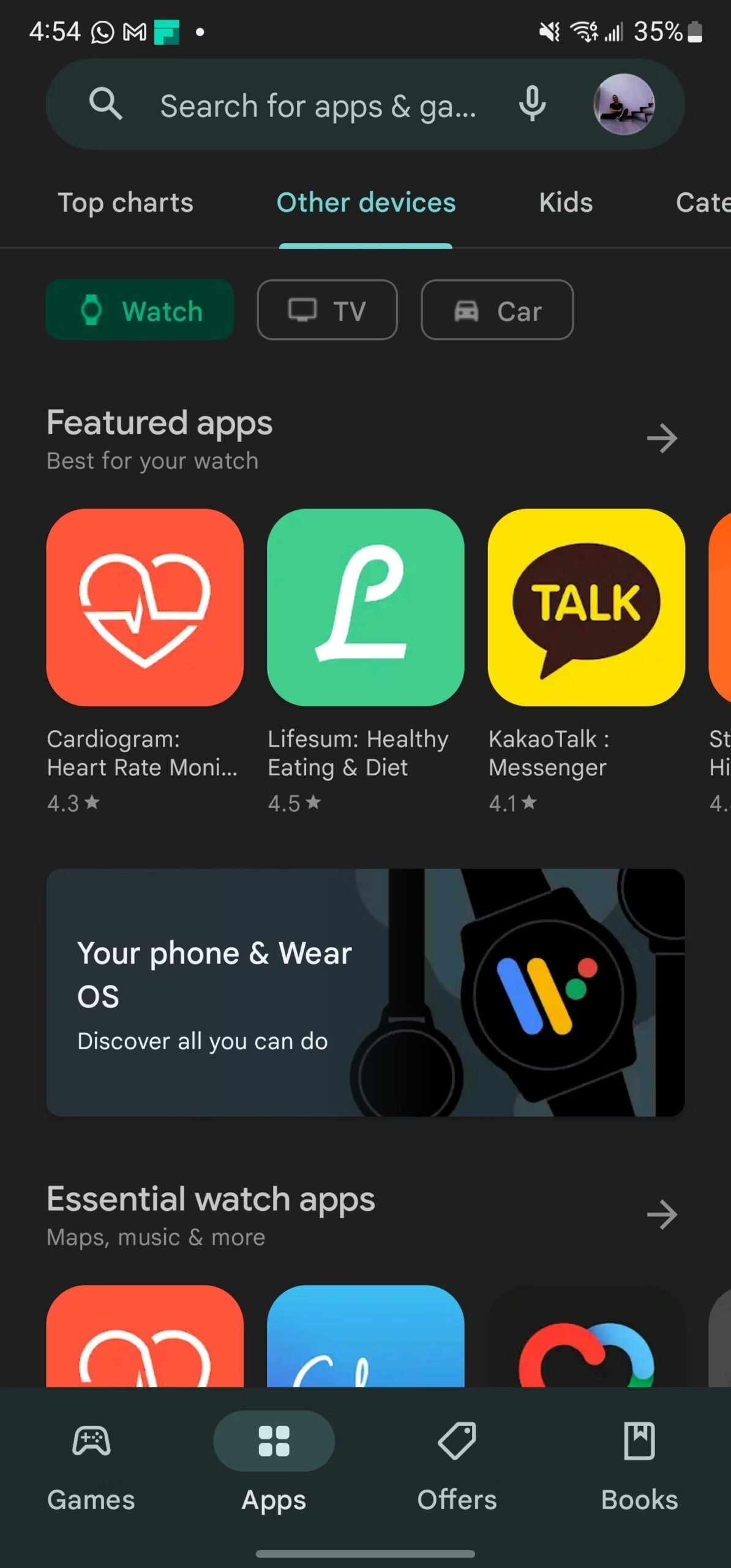**Caption**: This is a screenshot from a phone displaying an app store interface. At the top of the screen, you can see a search bar that reads "Search for apps at ga..." along with a microphone icon and a circle-shaped profile picture that is somewhat indistinct. Below, there are navigation tabs labeled: "Top charts," "Other devices," and "Kids." The "Other devices" tab is selected.

Within the "Other devices" section, three rectangular options are present: "Watch," "TV," and "Car." The "Watch" option is highlighted with a green background. Below, the section title "Featured apps best for your watch" is displayed, showcasing several app icons.

1. **Cardiogram: Heart Monitor** - This app icon features a red square with a white heart in the center and has a rating of 4.3 stars.
2. **Lifesum: Healthy Eating and Diet** - The icon is a green square with a white element and holds a rating of 4.5 stars.
3. **KakaoTalk: Messenger** - Displayed as a yellow square with a brown chat bubble and the word "Talk" in yellow font, it has a rating of 4.1 stars.

Towards the bottom, there's an illustration featuring three black smartwatches accompanied by the text: "Your phone and Wear OS, discover all you can do."